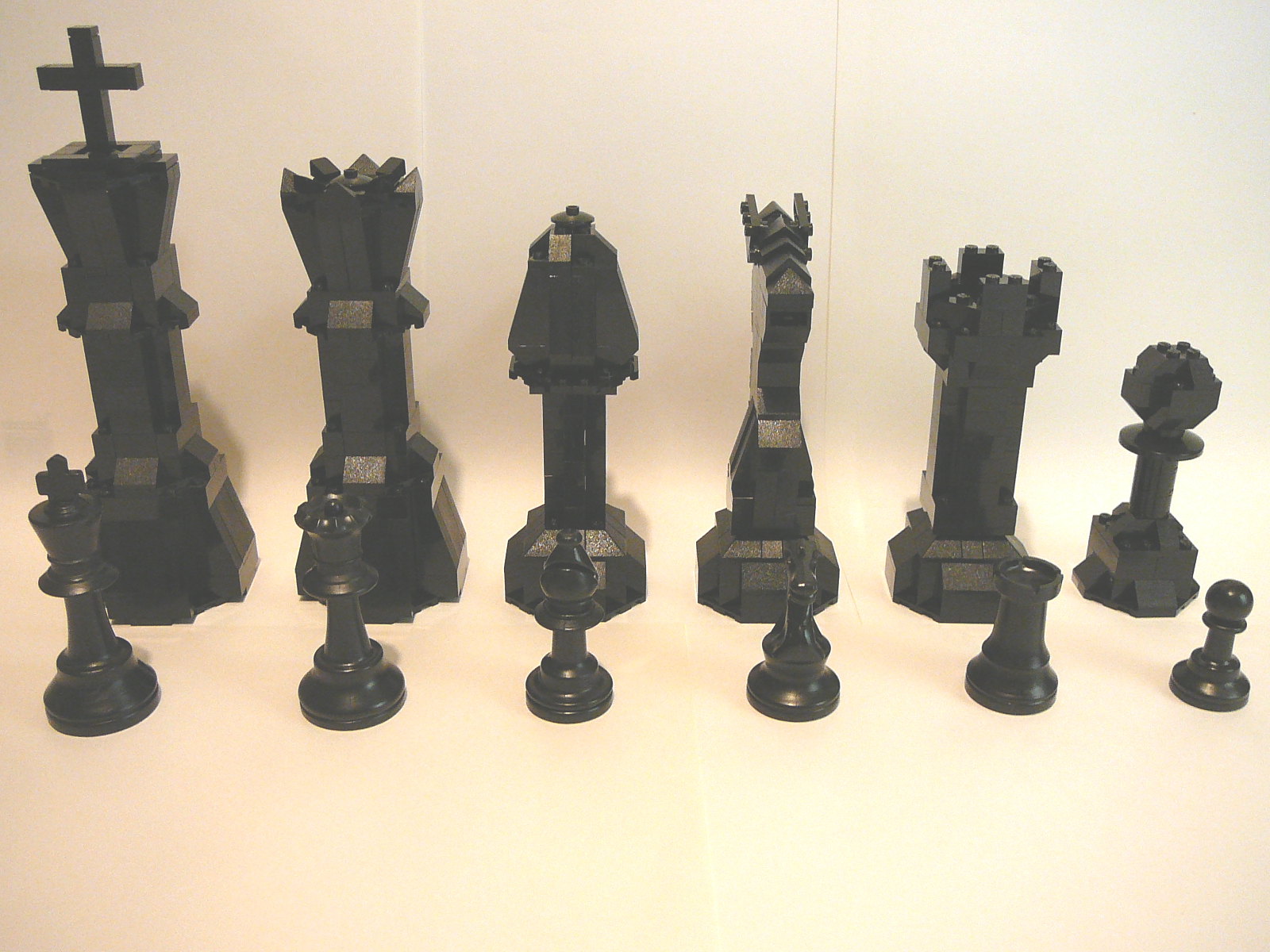This sepia-toned photograph depicts a comparison of traditional and Lego chess pieces, arranged meticulously on a beige surface against a beige background. The image features twelve chess pieces in total, organized into two horizontal rows of six pieces each. The front row, closer to the camera, contains smaller, traditional black chess pieces starting from the right with a pawn, followed by a rook, a knight, a bishop, a queen, and finally a king. The back row, made of larger Lego chess pieces, mirrors this arrangement with corresponding pieces: a pawn, a rook, a knight, a bishop, a queen, and a king. The monochromatic black of the chess pieces contrasts with the homogeneous beige setting, highlighting the distinct design differences between the traditional and Lego-made chess pieces.